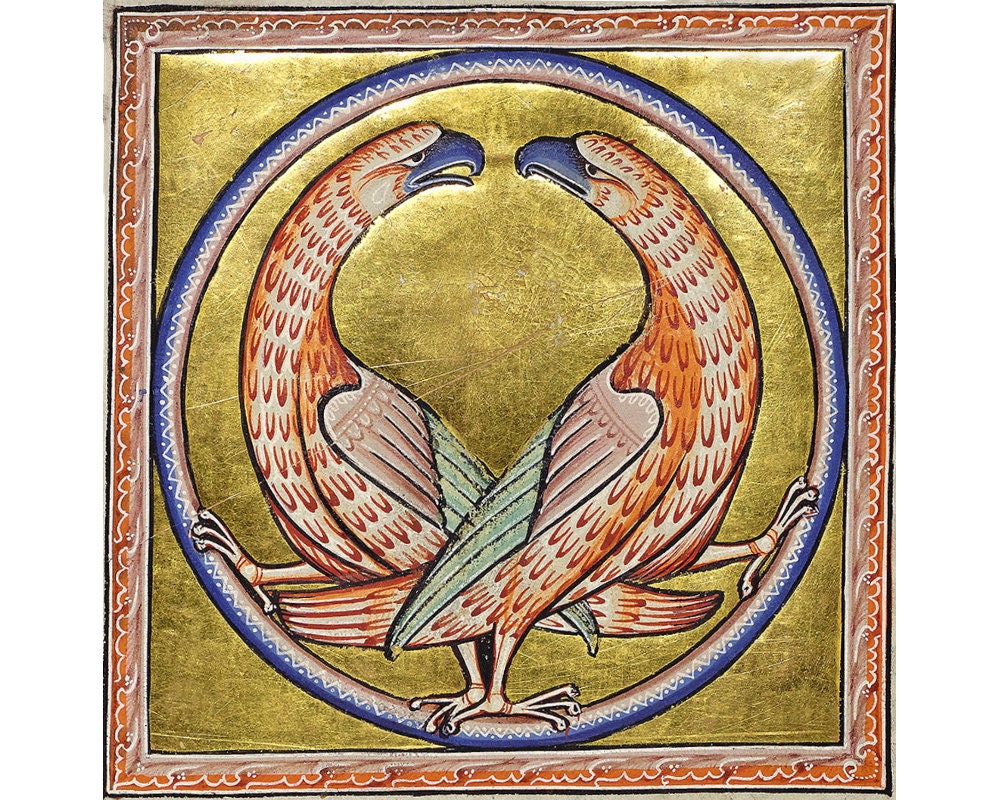This detailed illustration, possibly an artist's rendering or ancient color print, is framed by an intricate border. The border is layered with black and white lines, and features ornate red with what appears to be Arabic writing in white. The inner border is framed by another set of white and black lines. The primary background is a gradation from yellow to yellowish-brown, with reflective gold leaf areas adding a historic, ancient feel.

At the center of the image is a vivid blue circle, outlined in blue, with white squiggly patterns. Inside this circle, there are two stylized birds of prey, resembling long, tall, skinny eagles. These birds are facing each other, with their blue beaks close but not touching. Their eyes are yellow, and their feathers transition in color from dark brown to light brown and include a shade of light green on one wing. Each bird has one foot resting on top of the blue circle, while the other foot is positioned higher up, seemingly in a stance of mutual support or connection. The bird on the left has its beak open, suggesting an interaction or call, while the bird on the right remains silent, adding a dynamic element to their poised interaction. There are no other animals or people visible in this majestically detailed painting.